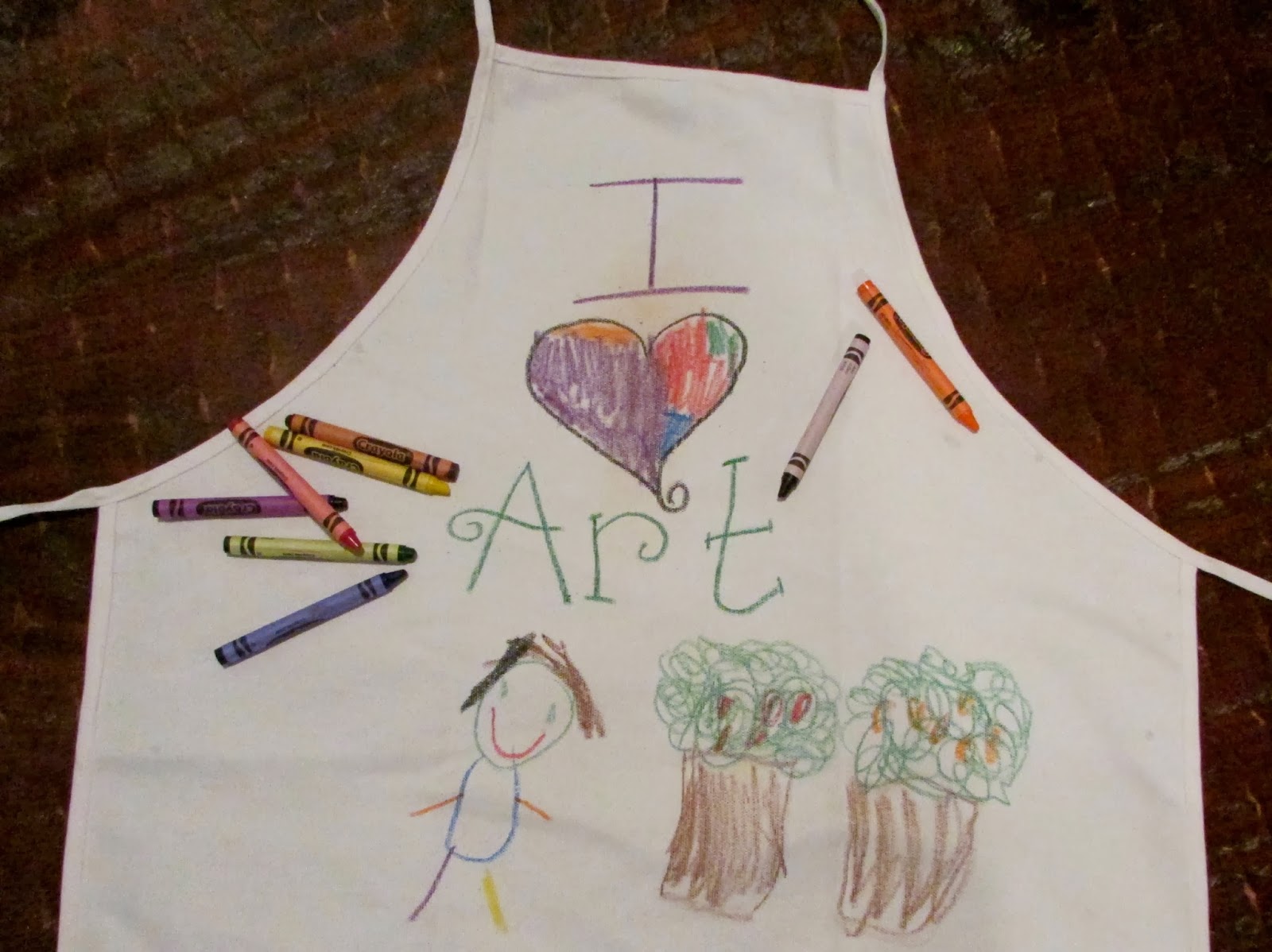The photograph depicts a charming do-it-yourself white apron, transformed into a colorful canvas by a child. The apron, initially plain, is now adorned with a heartfelt message, "I ♥ Art," where the heart shape is filled with a vibrant blend of purple, orange, red, green, and blue colors, accompanied by a whimsical squiggly line at its base that also appears under the letter 'A' in "Art." Below this declaration are expertly drawn depictions of two thick trees with swirly green leaves and a cheerful little boy. The boy is portrayed with brown and black hair, a beaming smile, blue eyes, and a delightfully mismatched outfit featuring orange arms, a purple leg, a yellow leg, and a blue body. Scattered across the apron are the child's crayons—orange, black, brown, yellow, red, purple, green, and blue—indicating the palette used for this creative endeavor. The whole scene is set against a red and brown background with white streaks, likely a table or floor, adding to the cozy, homey feel of the image.